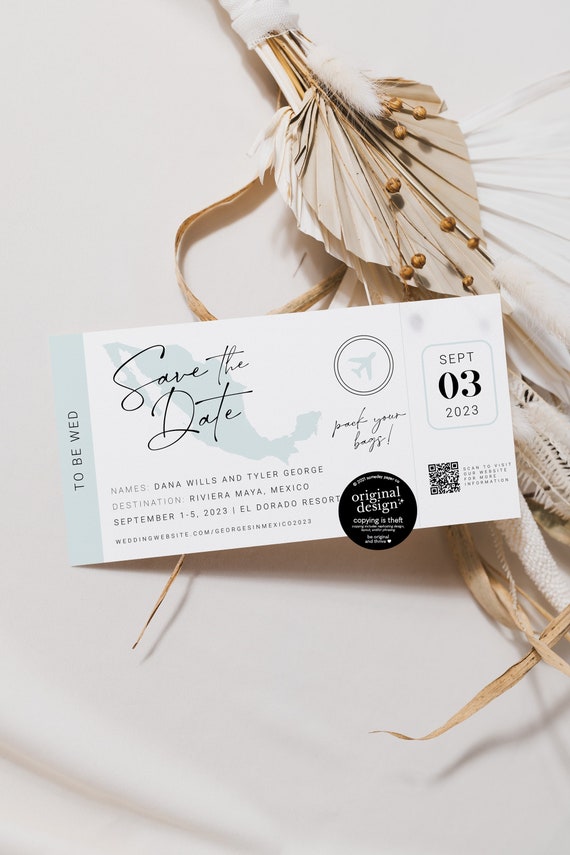The image is an artistic photo illustration with a white or ecru background featuring a dried botanical arrangement. The stems, wrapped in white cloth, come from the top middle of the image and fan out to the right, showcasing palm fronds, dried acorns, seed pods, and various grasses, all in natural tan and white hues. Superimposed over this arrangement is a "Save the Date" invitation card with an outline of Mexico. The card includes details of a destination wedding for Dana Wills and Tyler George, set to take place from September 1st to 3rd, 2023, at the El Dorado Resort in Riviera Maya, Mexico. It features a border on the left in pale blue, a circled airplane icon, a date of September 03, 2023, and the phrase "Pack your bags." There is also a QR code for more information, a watermark seal indicating original design, and mentions the wedding website. The overall aesthetic is shabby chic, with beige, floral, and pastel tones, creating a picturesque and aesthetically pleasing composition.